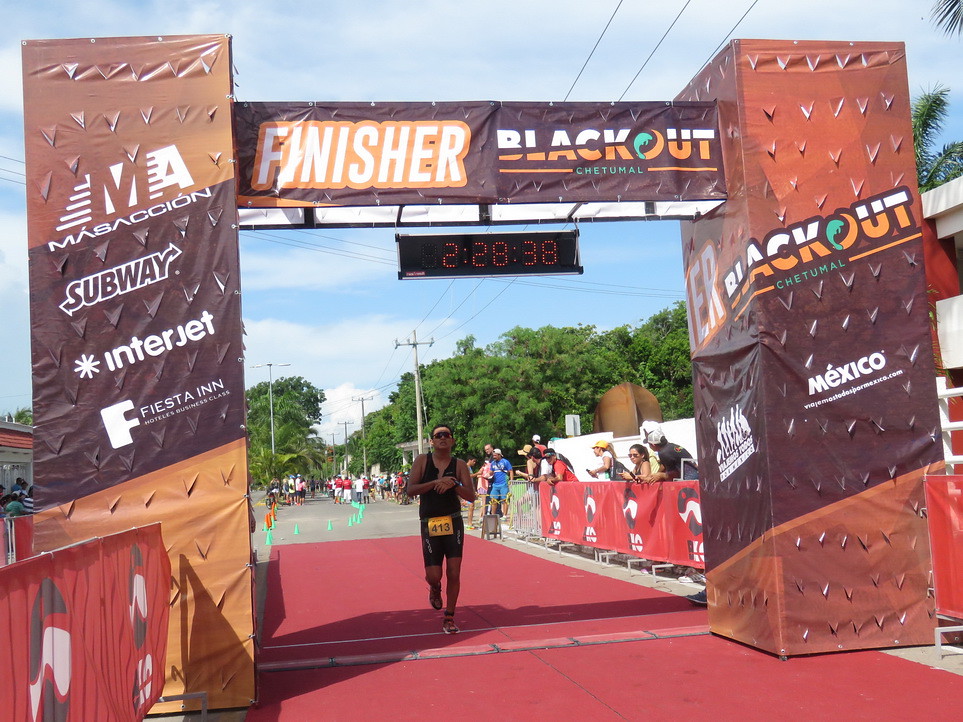The image captures a vibrant scene of a marathon finish line, set against a sunny blue sky. A male runner, dressed in a black tank top and shorts with the number 413, is crossing the finish line with an exhausted expression. A digital LED screen above him displays his completion time: 2 hours, 28 minutes, and 38 seconds. The finish line is flanked by two pillars adorned with the words "Finisher," "Blackout," and "Chetumal." Several sponsors, including Subway, Interjet, Fiesta Inn, and Mazaccion, have their logos displayed on red banners that drape the metal railings lining the course. Enthusiastic spectators are gathered on either side, cheering the runner's final steps on the red carpet. The background reveals green cones on the asphalt, separating the running course from the street, with rows of trees and power lines visible in the distance.